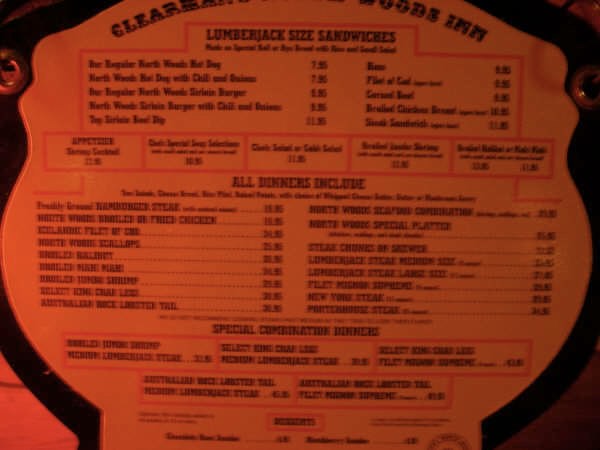The image features a restaurant menu cast in an orange hue, adding a warm ambiance to the presentation. The menu is framed by a distinctive black border with a wavy design, encasing a shape that is nearly circular but characterized by its undulating edges. The central background of the menu blends with the orange theme.

Prominently highlighted on the right-hand side, the menu boasts "Lumberjack Sized Sandwiches," though the detailed descriptions underneath are blurred beyond legibility. The pricing for these hearty sandwiches is clearly listed as $7.95, $7.95, $8.85, $8.85, and $11.35, indicating a range of options.

Sections of the menu outline various appetizers and salads, though specific details are obscured by the image quality. A note mentions that all dinners come with sides, though the list of these accompaniments is unreadable. 

In the dinner section, the following entrees are partially discernible: "steak chunks" followed by two unreadable words, "lumberjack steak," "filet mignon," and "New York steak," with a final entry for "porterhouse steak." A special combinations dinner is also mentioned, but the specifics are difficult to decipher due to the blurred text and a slight border over the image, adding to the challenge of reading finer details.